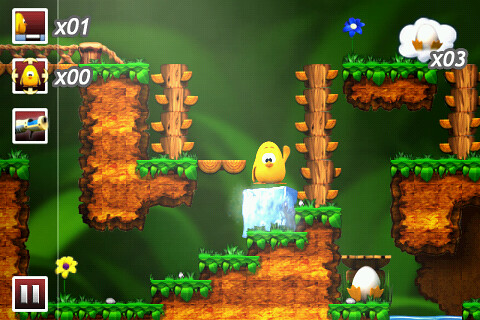In this vibrant screenshot from a video game, a small, cartoonishly stylized chick with bright, colorful feathers is prominently featured. The chick has two small black eyes set within a white circular patch, giving it an adorable, expressive appearance. It is depicted waving one of its tiny wings, seemingly interacting with the player. The game's setting appears to be a dense forest, distinguished by numerous green grass platforms and totem pole-like wooden structures that function as ladders. The backdrop is adorned with large, lush leaves, reinforcing the forest theme. On the screen, various game stats are displayed, including icons of the chick and corresponding numerical values, contributing to the immersive gaming experience.